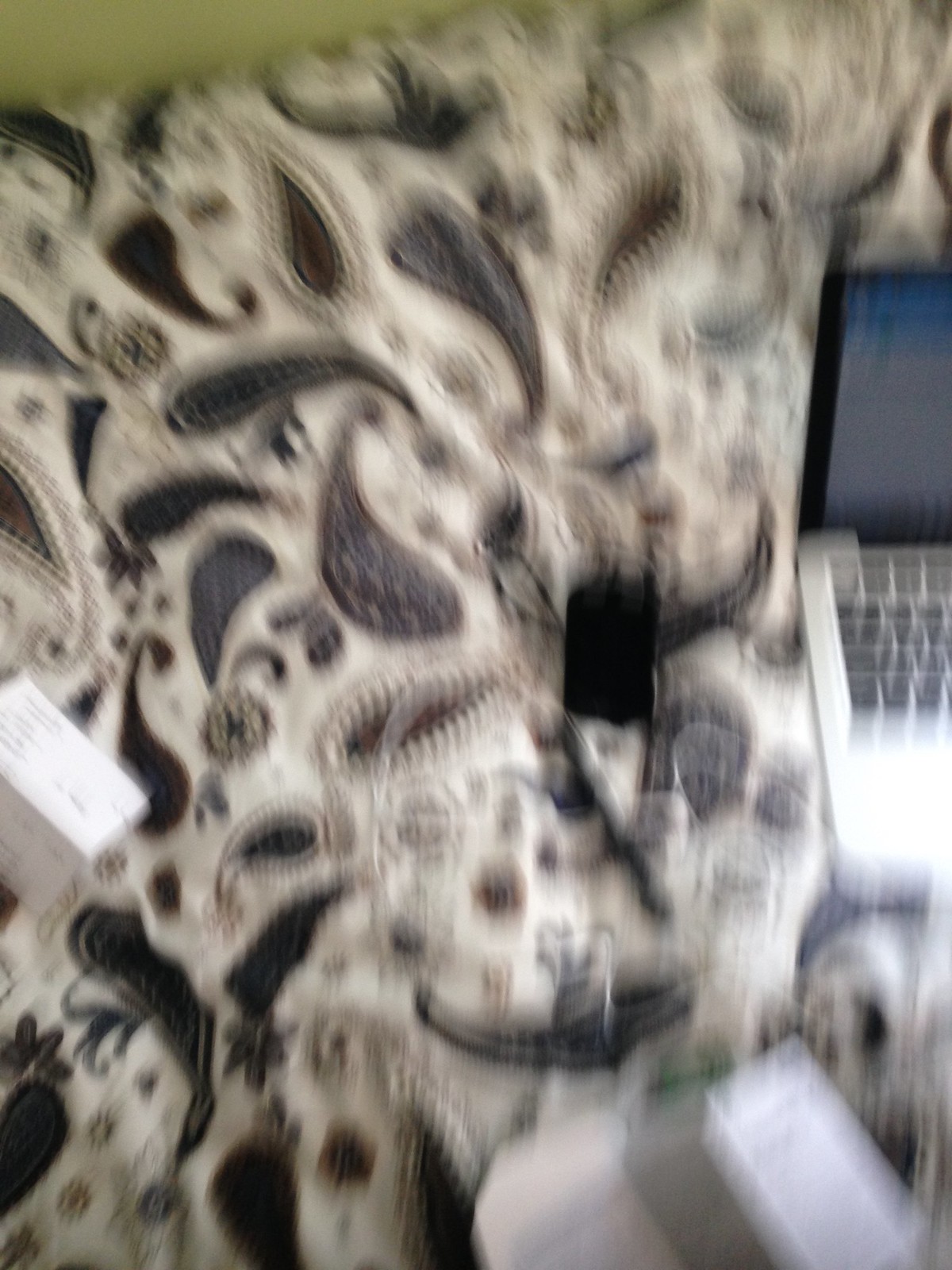This image appears blurred due to motion, resulting in a somewhat indistinct overall appearance. However, a few elements are discernible:

- On the right edge, a portion of a silver laptop computer with a black bezel is partially visible. The screen is open, showing the first few rows of keys on the keyboard.
- The majority of the background features a large Paisley-patterned bed comforter.
- Near the laptop, there is a black object, the specifics of which remain unclear due to the blurriness.
- On the left side of the comforter, there is a white box.
- At the bottom right, a folded piece of white paper can be seen.

This composition suggests a cozy, possibly busy, area where someone might be working or relaxing.